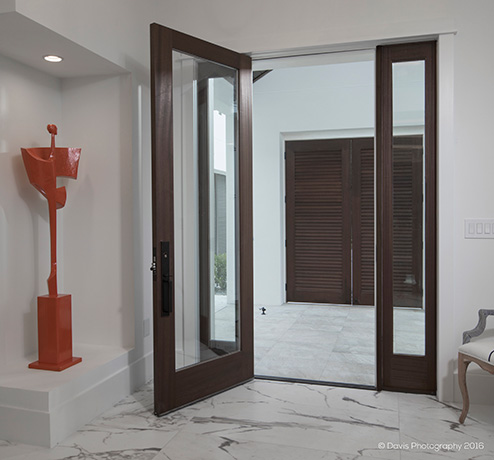The image depicts an elegant entryway bathed in white with a modern, minimalist aesthetic. The room features pristine white walls and a white ceiling, with the floor showcasing a sophisticated blend of white, gray, and black marble. To the left, a white platform supports a striking red artistic sculpture, illuminated from above by a discreet can light. A light switch with three buttons is mounted on the adjacent wall. On the right-hand side, a small chair with brown legs, a gray handle, and a white cushion accented by a black stripe sits partially in view. The open door reveals a breezeway area, leading to an exterior with two dark chocolate-stained doors and a continuation of the marble flooring. In the bottom right corner of the image, the watermark "Davis Photography 2016" is visible, signifying the photographer's copyright. The sophisticated setting evokes the ambiance of a high-end spa or a luxurious hotel rather than a conventional office space.